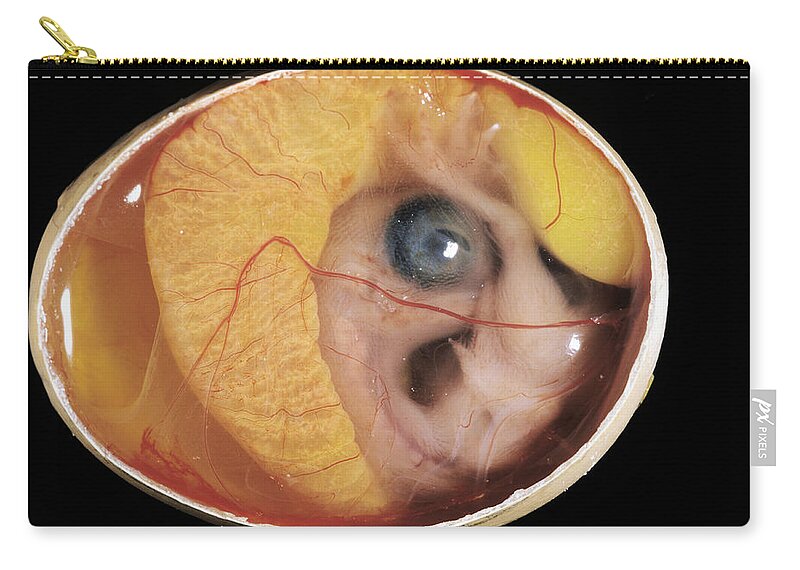The image depicts a rectangular hand purse or change purse measuring about five inches wide and three inches high. The purse features a gold zipper at the top with the tab positioned on the upper left. Below the zipper, a white dotted stitching line crosses horizontally against a black fabric background. The standout design element on the purse is an intricate and somewhat strange depiction of a cut-open egg embryo. The image captures a baby bird, likely a chicken, with a large blue eye and pinkish skin, curled up with its feet tucked over its head. The egg's interior reveals yellow yolk surrounded by tiny red veins and blood vessels, contributing to a realistic portrayal of an embryonic development. There is also a small tag on the lower right side of the purse that reads "PX pixels." The entire design offers a highly detailed and surreal aesthetic for a hand purse.